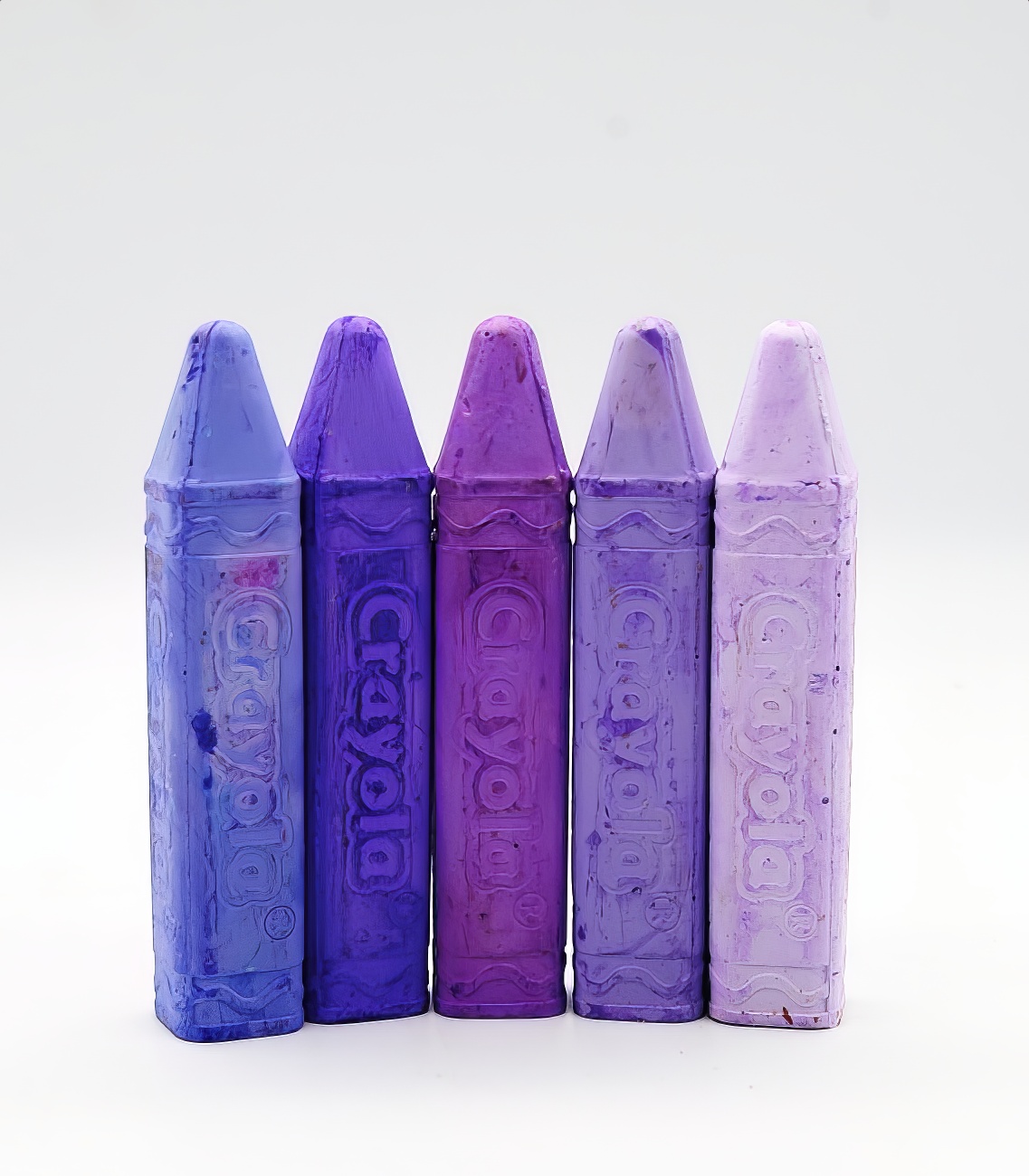The image depicts five pieces of Crayola chalk intricately crafted to mimic the iconic shape of Crayola crayons, with a pointed top and rectangular bodies. Captured in a studio setting against a white background, slight shadows outline the chalk. The chalk is arranged from left to right in varying shades of blue and purple hues. From left to right, the colors transition from a light periwinkle blue, a deep indigo, a vibrant purple, a powdery lavender, to a very light lavender. Each piece of chalk is engraved with the Crayola logo and features a distinctive squiggly line reminiscent of crayon labels. Though the chalk appears new, subtle dings and dents suggest they've been jostled with other colors, as indicated by faint, different-colored streaks on their surfaces.